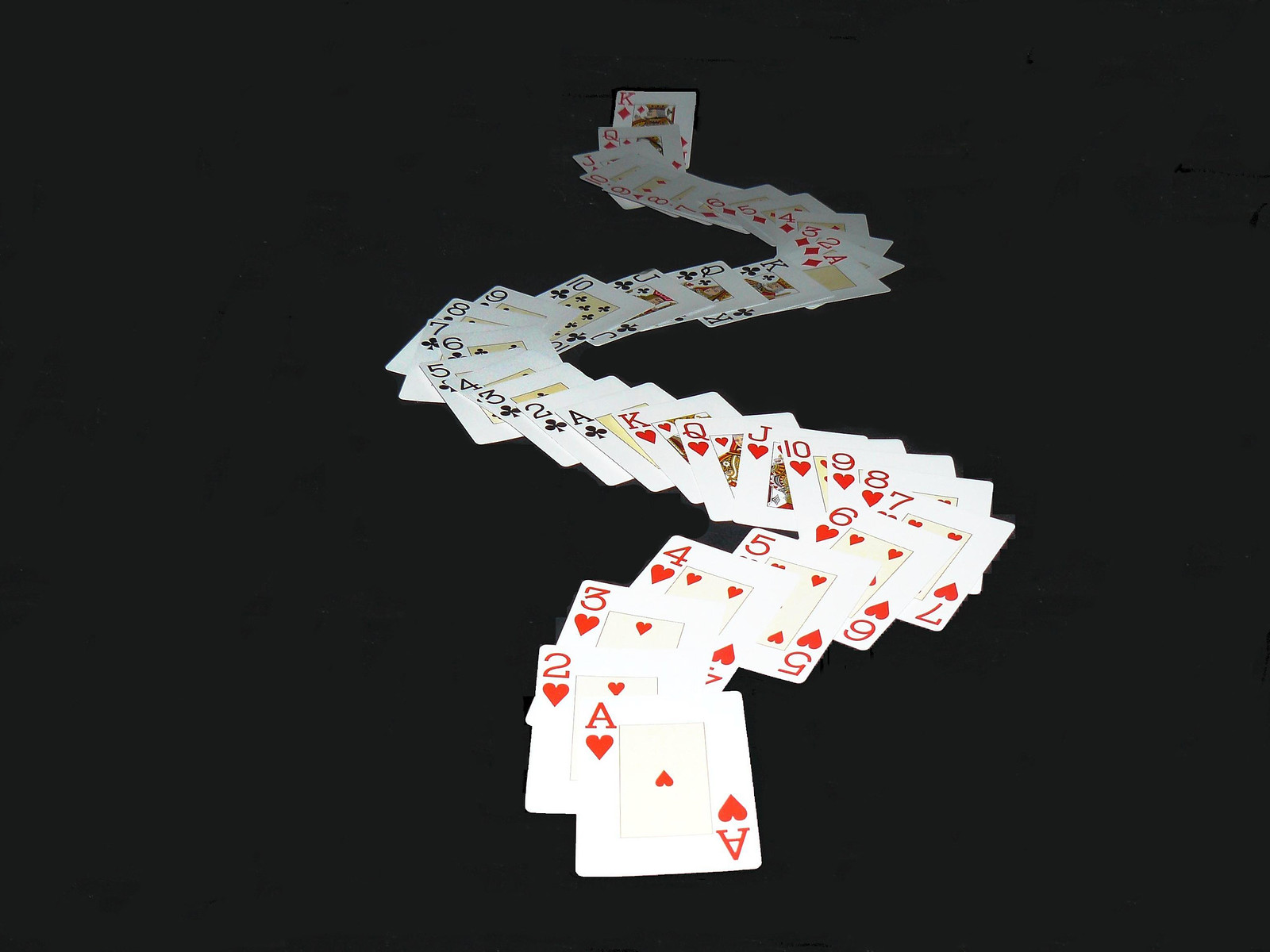The image showcases a black background, possibly a tablecloth or a table, against which a full deck of playing cards is prominently displayed. The cards are laid out in a single, continuous line that begins at the middle bottom of the image with the Ace of Hearts. The line curves elegantly to the right before sharply turning to the left, ascending as it transitions into the suit of Clubs. This pattern continues with another sharp right turn leading into the red Diamonds, and finally, another left turn before straightening out and once again traveling upward through the middle of the image. The suits are shown in sequence: Hearts, Clubs, and Diamonds, each represented by its full complement of cards from Ace through King. The vibrant red of the Hearts and Diamonds contrasts beautifully with the black Clubs, creating a striking visual effect against the backdrop.